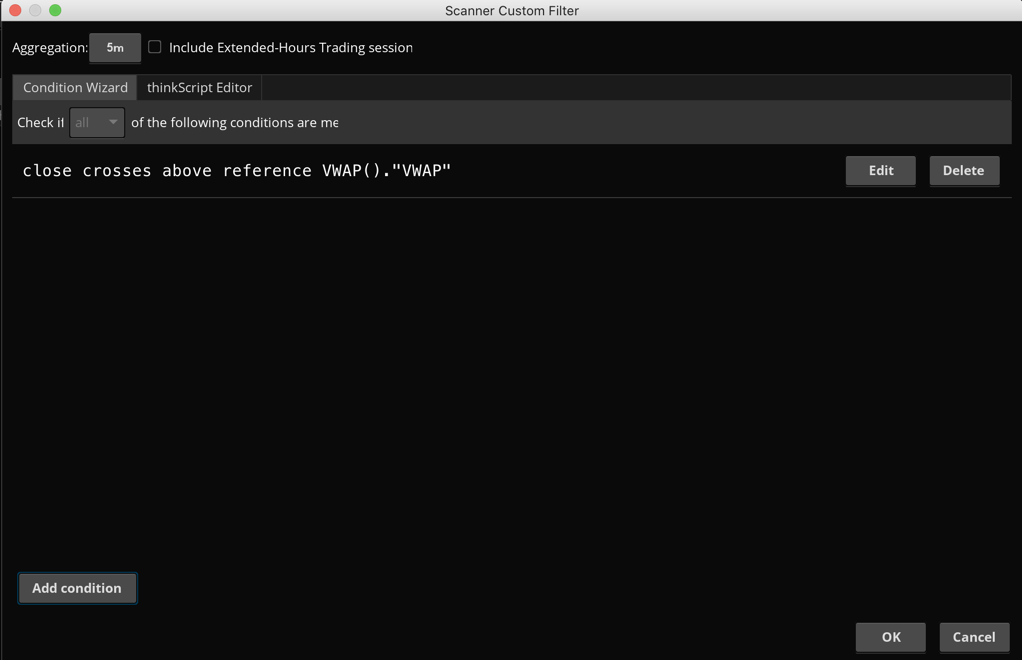The image is a screenshot showcasing a computer interface with a predominantly black background. At the very top, there is a thin, light gray bar labeled "Scanner Custom Filter." Below this, the first line displays the word "aggregation" followed by "5M." 

Next to this, a small square is ticked, with white text reading "Include extended hours trading session." Beneath this, the screen features "Condition Wizard" and "Think Script Editor" options. 

Under these options, there is a section with "All is defaulted" accompanied by a dropdown arrow. The text "Of the following conditions are" is partially visible, with the rest of the sentence truncated and beginning with the letters "M-E."

Following this, there is a script-like text that reads, "close crosses above reference VWAP ()." In quotation marks is the term "VWAP." To the far right of this line, there are two buttons labeled "Edit" and "Delete." 

The remaining screen area is primarily black and empty. At the bottom left, there is a button labeled "Add Condition," while the lower right corner features "OK" and "Cancel" buttons.